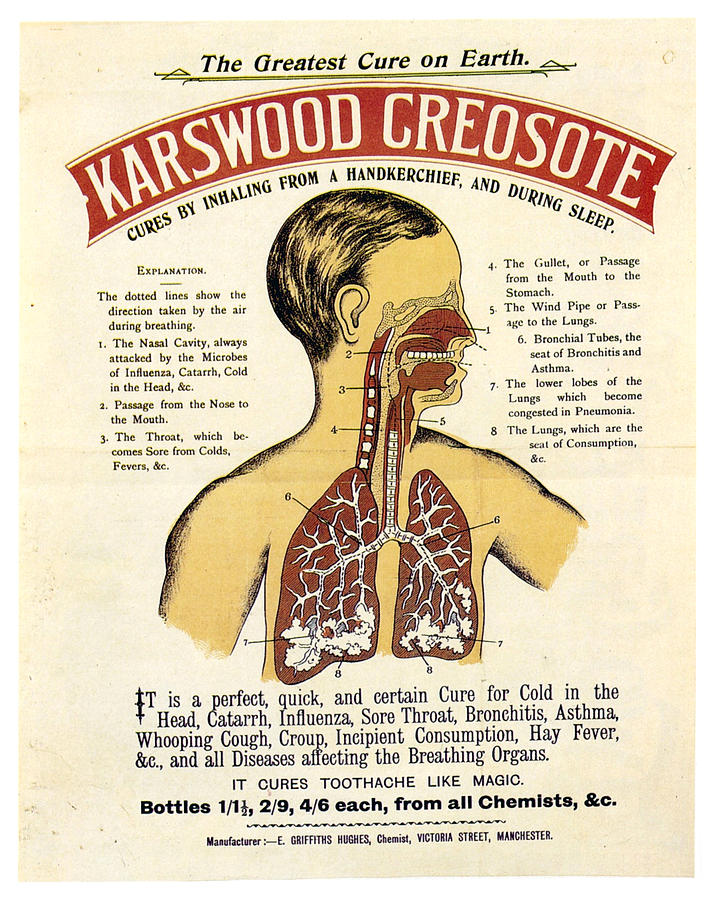This image displays an antiquated advertisement, likely from the early 1900s, proclaiming "The Greatest Cure on Earth." It prominently features a curved red banner with the product name, "Carswood Creosote." The poster describes how the remedy, which can be inhaled from a handkerchief or during sleep, functions. Central to the image is a detailed anatomical diagram of a man showcasing the respiratory system, from the mouth and teeth down to the lungs. Surrounding the illustration is extensive text that elaborates on the product's effectiveness. It claims to be a quick, perfect, and certain cure for a multitude of respiratory ailments, including cold in the head, catarrh, influenza, sore throat, bronchitis, asthma, whooping cough, croup, incipient consumption, and hay fever. Additionally, it touts its magical ability to relieve toothache. The advertisement concludes with pricing information and where the remedy can be purchased.